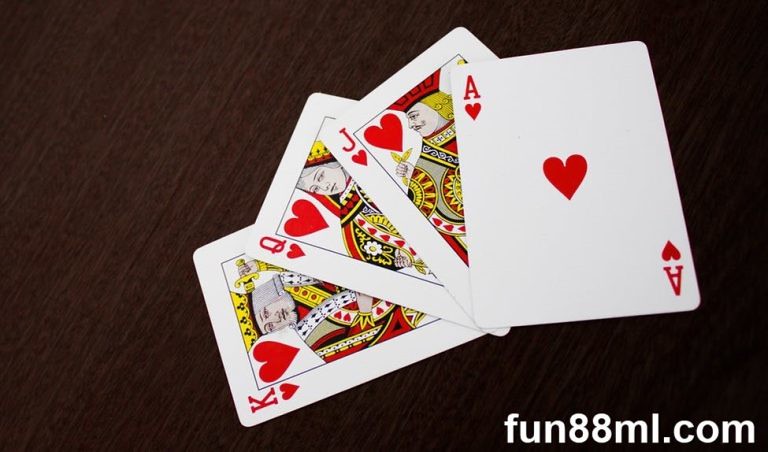The image features a meticulously arranged spread of four playing cards from a classic deck. The cards include the King of Hearts, Queen of Hearts, Jack of Hearts, and the Ace of Hearts, all unified by their strikingly rich red hue. The King of Hearts stands out in his regal attire, adorned with a golden crown, a short chin-length haircut, a cleft chin, and a gold, red, and white outfit. He holds a sword behind his head, reinforcing his authoritative presence.

The Queen of Hearts, though partially obscured, is bedecked in a sumptuous ensemble of gold, black, and red, and wears an intricate gold head cover. The Jack of Hearts, also known as the Joker in this context, sports a flamboyant red hat accented with black and gold, holding an unidentified object in his hand, with an ornate insignia adding to his whimsical yet elegant appearance.

The Ace of Hearts is minimalist in design, featuring a prominent red heart in the center and smaller red hearts positioned under the letter 'A' in two corners of the card. Each card reflects the traditional and timeless designs typical of a standard playing deck, emphasizing both artistry and function.